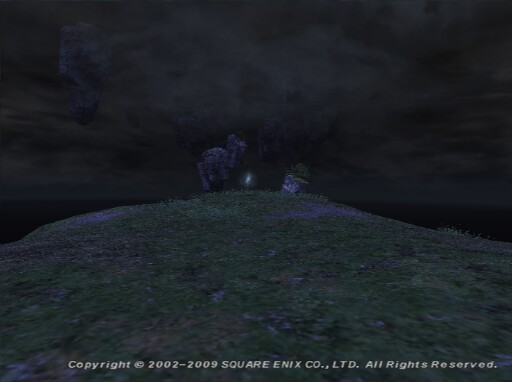In this dark and ominous video game scene, we find ourselves at the top of a dimly lit hill covered in sparse grass. The background is dominated by an intensely dark and stormy sky, adding to the sense of foreboding. In the middle of the hill, a faint and small white light offers the only source of illumination. To the left of this light stands an indistinct creature that appears to have a dinosaur-like form. On the right side of the light is an object whose nature is unclear; it looks like it could be a tilted gravestone. At the bottom of the scene, text reads, "Copyright 2002-2009, Square Enix Co., Ltd., All Rights Reserved."